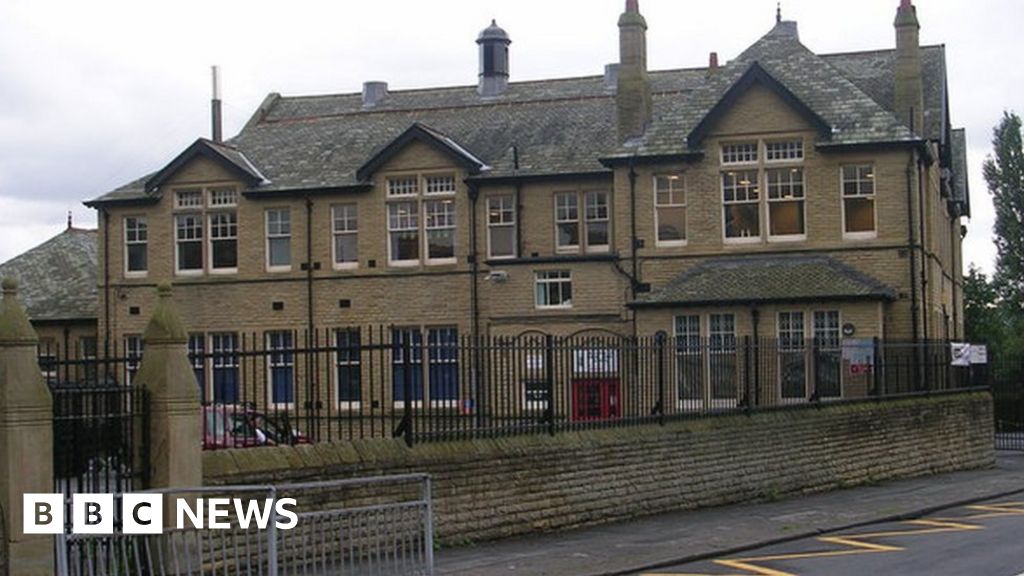The image shows a large, two-story brown building with numerous windows on both levels, some of which are open while others are closed. The building features a black shingle-like roof topped with several chimney-like structures. In the foreground, there is a diagonal sidewalk and street leading toward the bottom right corner, flanked by a stone wall and black wrought iron fence. A parked car is visible behind the fence on the left side. The lower left corner of the image contains a watermark with the text "BBC" in white blocks followed by the word "News." The sky is overcast with faint whitish-gray clouds, and a tall tree stands to the far right of the frame. A red doorway with an illegible white sign above it is noticeable on the building's facade, hinting at the building's possible function as a medical center, school, or business.